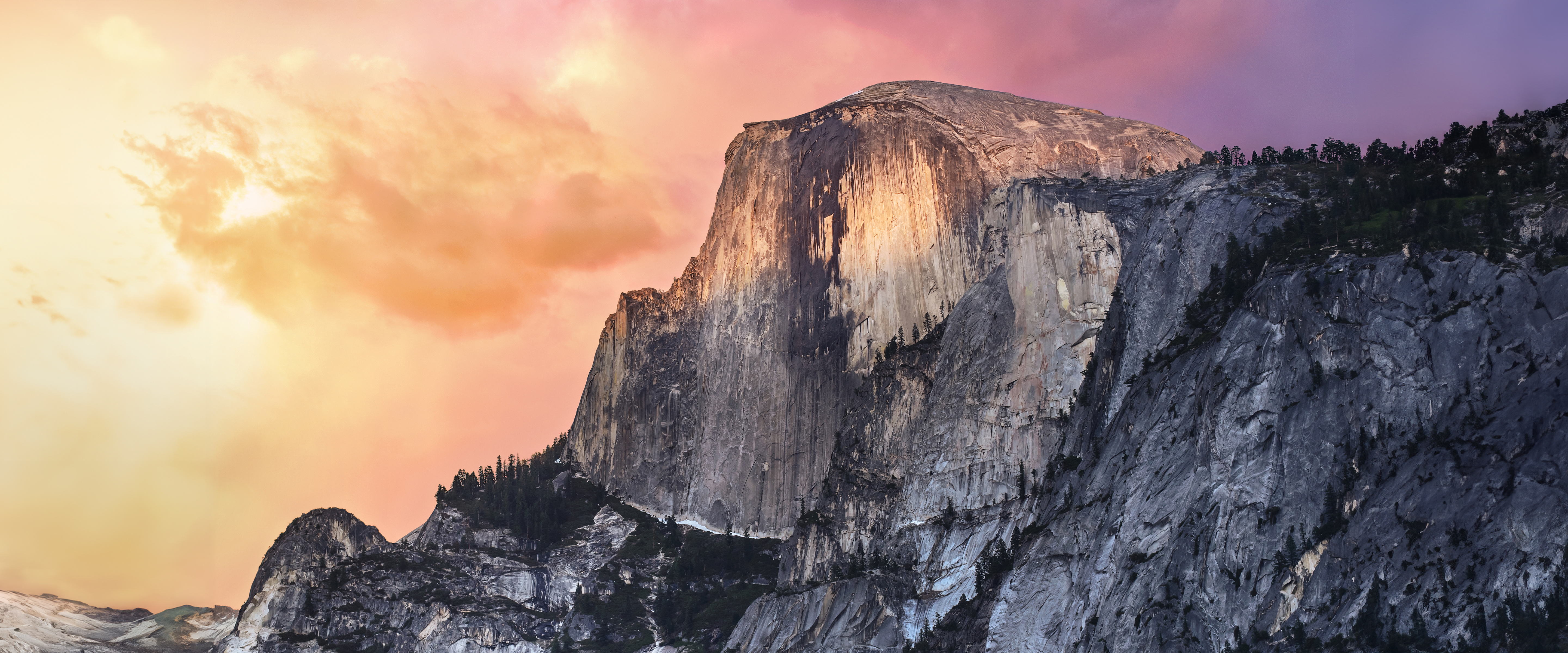The outdoor image captures a dramatic sky filled with clouds of varying colors. On the left side, the sky is tinted with a warm orange hue, which seamlessly blends into a large, puffy white cloud at the center, also tinged with shades of orange. As the view moves towards the background, the sky transitions to a melon color and continues through a gradient of pink, mauve, and finally purple on the right side. Beneath the clouds, there's a stratified rock formation. On the left, the rock level is lower, gradually rising towards the center where it peaks, and then tapering off again as it extends towards the purple-tinted sky. The rock surface is rugged, featuring numerous crevices and jagged outcrops that add texture and depth to the landscape.